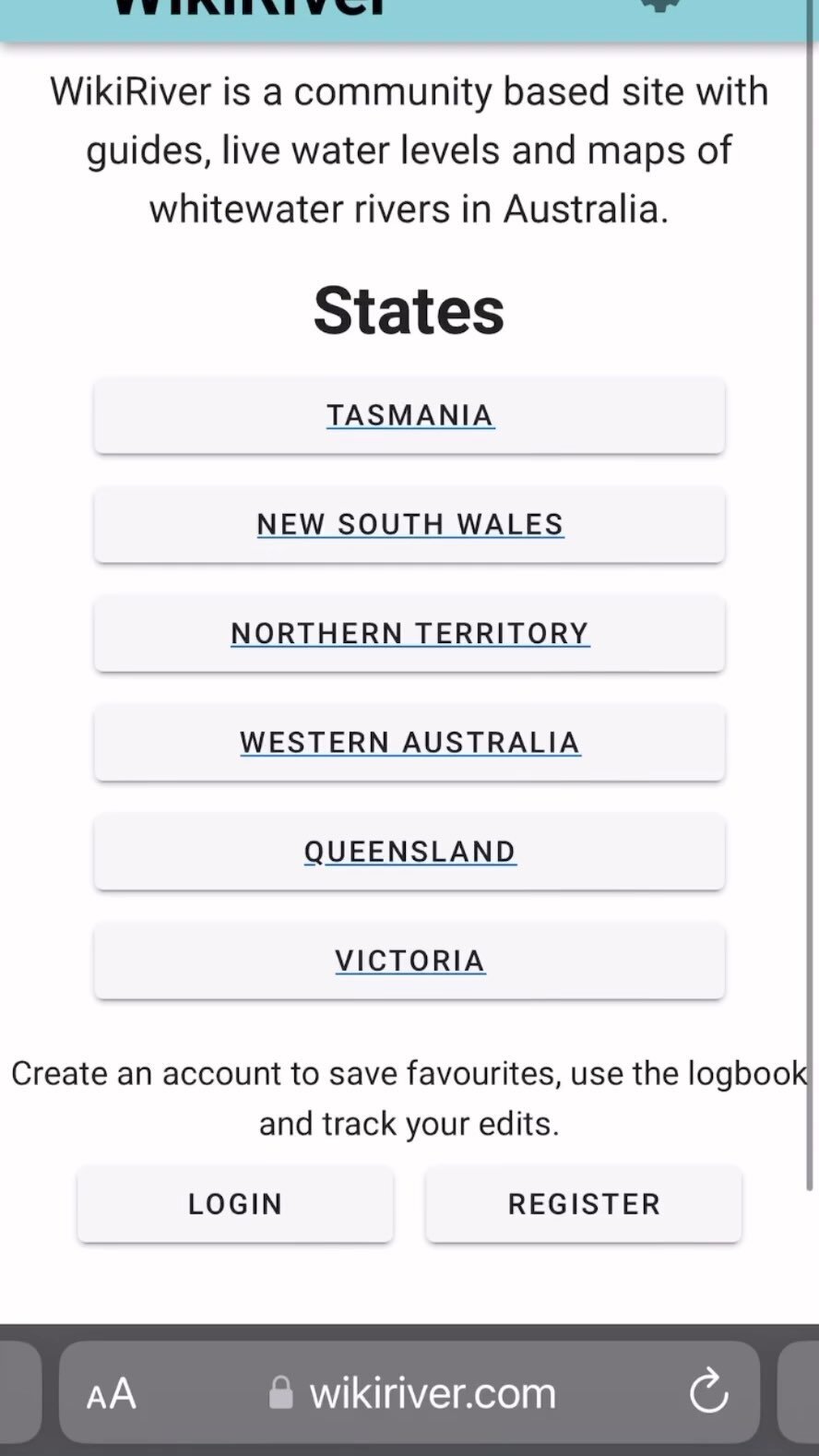The screenshot appears to be taken from a mobile phone screen featuring the Wicke River community site, which provides guides, live water levels, and maps of whitewater rivers in Australia. The interface has a blue border at the top and a white background featuring the main content area.

At the top of the white background, there's an introduction describing the site's purpose: "Wicke River is a community-based site with guides, live water levels, and maps of whitewater rivers in Australia." Below this, there is a list of six states, each represented by clickable rectangular buttons with underlines. The states listed are Tasmania, New South Wales, Northern Territory, Western Australia, Queensland, and Victoria.

Further down, the white background features a prompt encouraging users to create an account in order to save favorites, use the logbook, and track their edits. This section is accompanied by two rectangular buttons: one labeled "Login" and the other "Register."

At the very bottom of the screen, there is a gray background. In the far left corner of this gray section, there are two 'A' icons, one smaller than the other, followed by a padlock icon and the website address "wickeriver.com". On the far right side of this gray section, there appears to be a refresh icon. Additionally, a black line is visible along the right side of the screen.

Overall, the screenshot captures the layout and functionalities of the Wicke River site, including navigation buttons for different states in Australia, account login/register features, and some site footer elements.